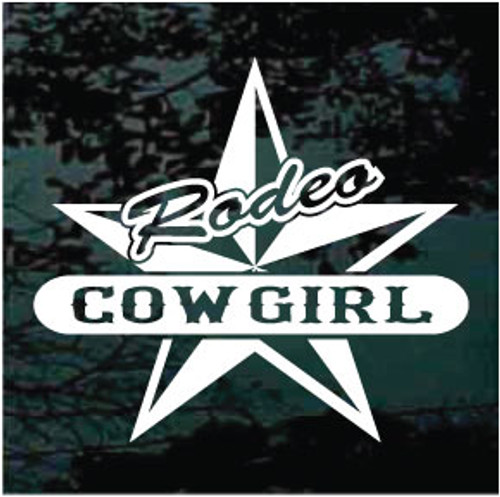The image displays a detailed, monochromatic rodeo cowgirl logo set against a very dark, nighttime scene. The background, shrouded in shadows, features tree branches and leaves silhouetted against a dim, overcast sky. Central to the image is a distinctive white and black, five-pointed star where each point alternates between solid white and transparent, allowing the dark backdrop to peek through. Inscribed diagonally across the top of the star in cursive text is the word "Rodeo," slanting upwards to the right. Below it, within an elongated oval or pill-shaped white box, appears the word "Cowgirl" in clear, capital letters. The intricate design of the logo, combined with the strikingly dark environment, creates a compelling visual contrast.